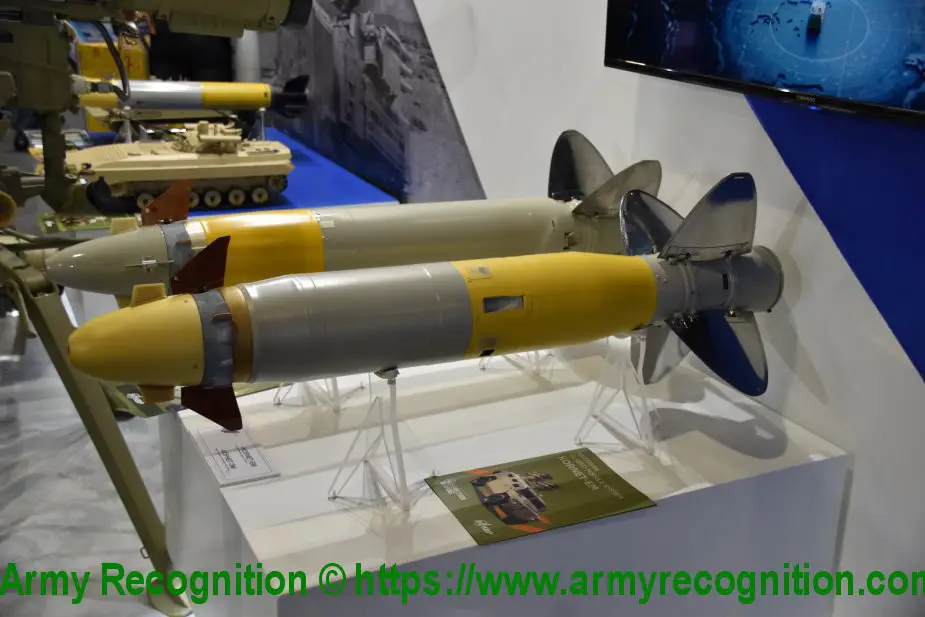The image captures a detailed museum display featuring small rockets or missiles, each approximately three to four feet in length. The missiles are predominantly silver with alternating yellow and gray sections, comprising yellow cone heads, gray centers, and gray fins. One of the warheads is distinguished by a green body with a yellow neck. These rockets are mounted on clear plastic stands, positioned on a white display platform that includes a partly legible pamphlet and a descriptive plaque. In the background, prominent features include a miniature tank model to the upper left, a black and white mural possibly depicting a building, and a TV screen displaying information. The bottom of the image is overlaid with bright green text reading "Army Recognition Copyright HTTPS://www.armyrecognition.com," suggesting a focus on military technology. The overall scene is set against a flat concrete ground, indicating the display area is part of an organized exhibition space.